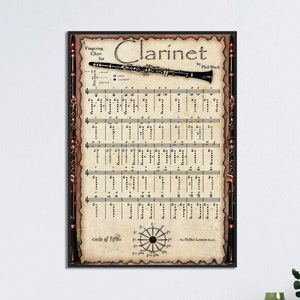The image depicts a framed poster about the clarinet, prominently featuring the word "Clarinet" at the top in black lettering. Below the title, a black clarinet illustration stretches horizontally from left to right. The black frame incorporates clarinet motifs on both the right and left sides. The poster is detailed with five rows of schematic dots, some filled and some not, likely indicating finger placements for different notes on the instrument. At the bottom, there's a circular diagram with a black dot in the center, radiating lines, and flanked by text that is too small to read clearly. The overall background of the poster is white, set against what seems to be a light-colored wall, possibly light blue. Despite being a small and blurry image, the setting appears well-lit, hinting that it might be displayed in a home environment. There's a vague glass or lamp object visible at the bottom, but details are indistinct.